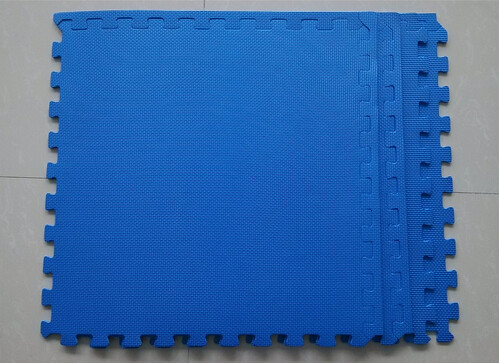This image showcases a detailed close-up of four large, dark blue foam tiles designed for interlocking, detachable flooring. Each tile features tapered, puzzle-like teeth along its edges, allowing them to fit and lock together seamlessly. These tiles, commonly used for play areas or garage floors, are stacked neatly on top of each other, with the first one fully visible and partially covering the others, highlighting the interlocking teeth. They cast subtle shadows on a gray tiled floor below, characterized by thin grout lines and light gray specks. The photograph is brightly lit, emphasizing the vivid blue color and the texture of the foam tiles.